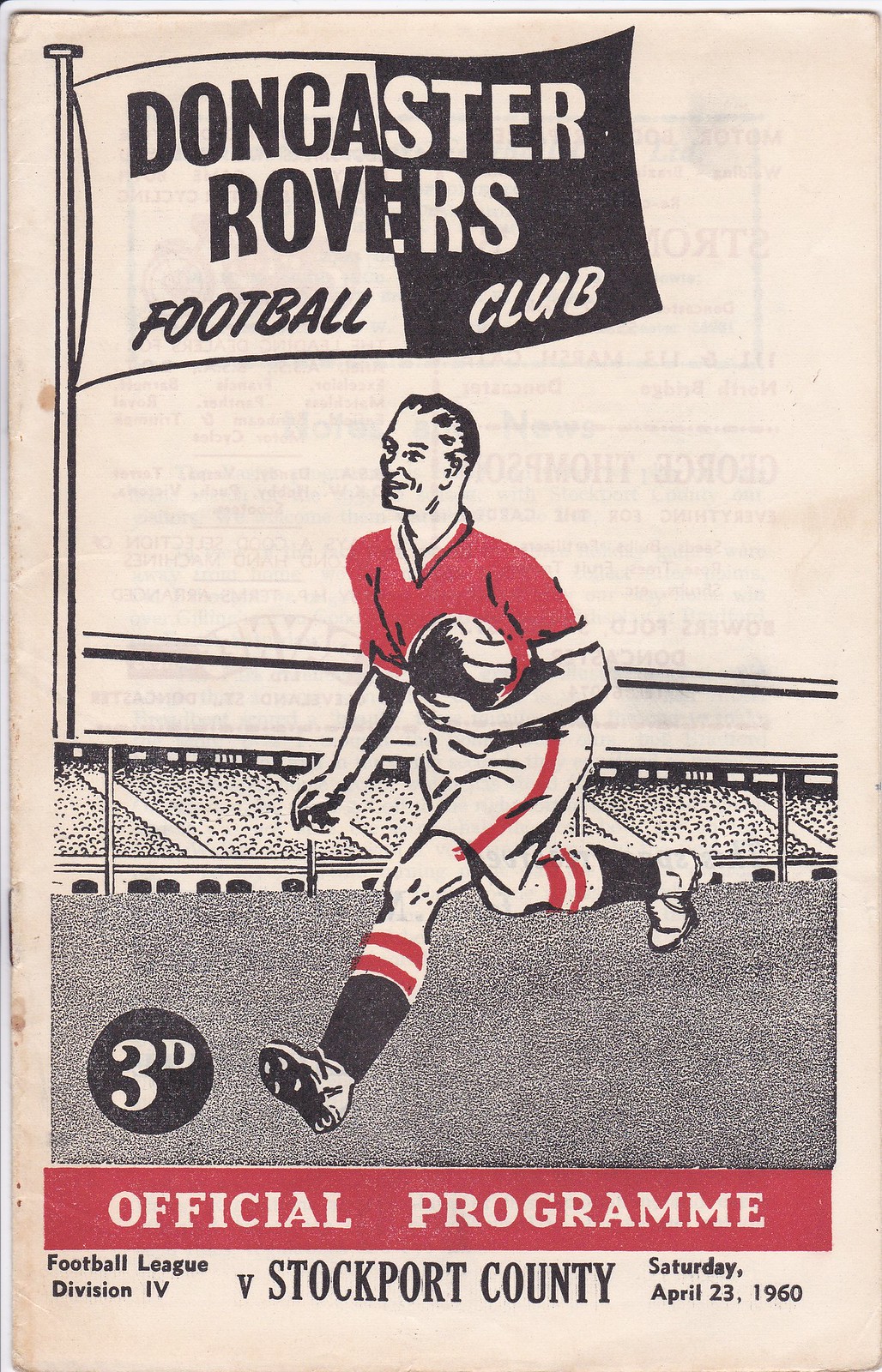This image is the cover of an old, slightly faded soccer program from April 23rd, 1960, featuring the Football League Division 4 match between Doncaster Rovers Football Club and Stockport County. The background is the original white color of the paper, with hints of a pink tint and visible stains and creases, suggesting its age. At the very top of the cover, there's a distinct black and white flag design with 'Doncaster Rovers Football Club' written on it, where the text color contrasts with the flag's halves. This flag is attached to a drawn flagpole that connects to an audience seating area represented by squiggly lines to indicate a full crowd. Below this is a large picture of a soccer player running with a soccer ball. The player is centrally located and is depicted wearing a short-sleeve red shirt, white shorts with a red stripe on the sides, black socks with white and red stripes at the top, and soccer cleats. At the bottom left of the cover, it reads "3D" and underneath, it says "Official Program." Further down, it details "Football League Division 4 versus Stockport County Saturday April 23rd 1960." The color palette includes white, tan, black, and red, enhancing the vintage feel of the program.